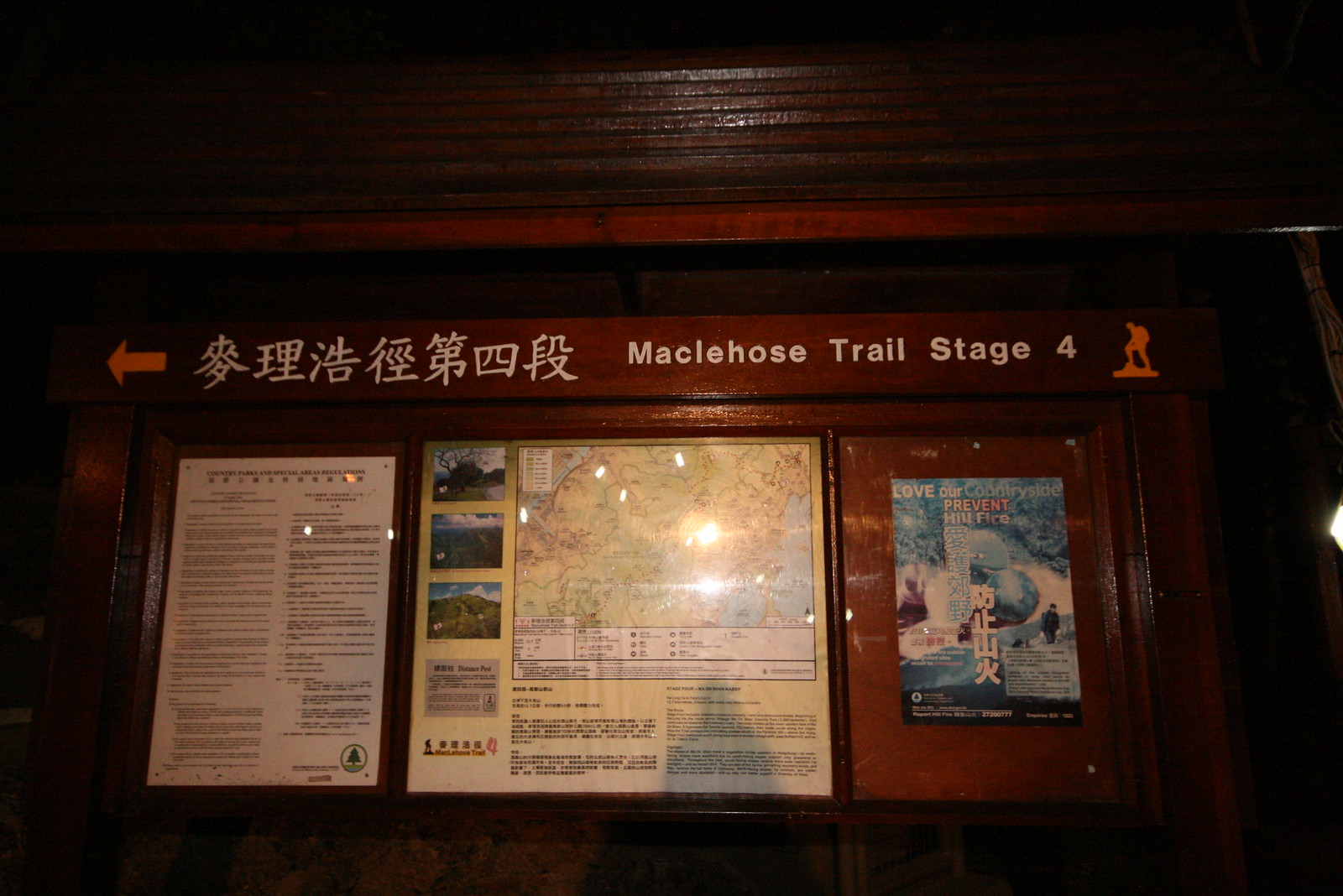The image depicts a large, dark stained and grainy wooden signboard positioned on a trail, likely at the entrance or a significant point of the Macklehose Trail Stage 4. The scene is either captured at night or under poor lighting, as indicated by scattered light reflections on the wood and glass cases. Prominently displayed at the top of the sign is an orange arrow pointing left, accompanied by white Chinese text and the English phrase, "Macklehose Trail Stage 4." In the top right corner, there is an orange silhouette of a hiker.

Beneath the main signage, three sections enclosed in glass are discernible due to the light reflecting off the glass surfaces. On the far left, there is a white sign with black text, which appears to have two columns, possibly with English on one side and Chinese on the other. The central section features a map, complete with photographs of points of interest along the trail, and text detailing various aspects of the path, including a dotted line indicating the trail route. On the right, there is a vibrant poster predominantly featuring blue, bearing the message, "Love Our Countryside, Prevent Hill Fire," aimed at promoting environmental awareness and fire prevention.